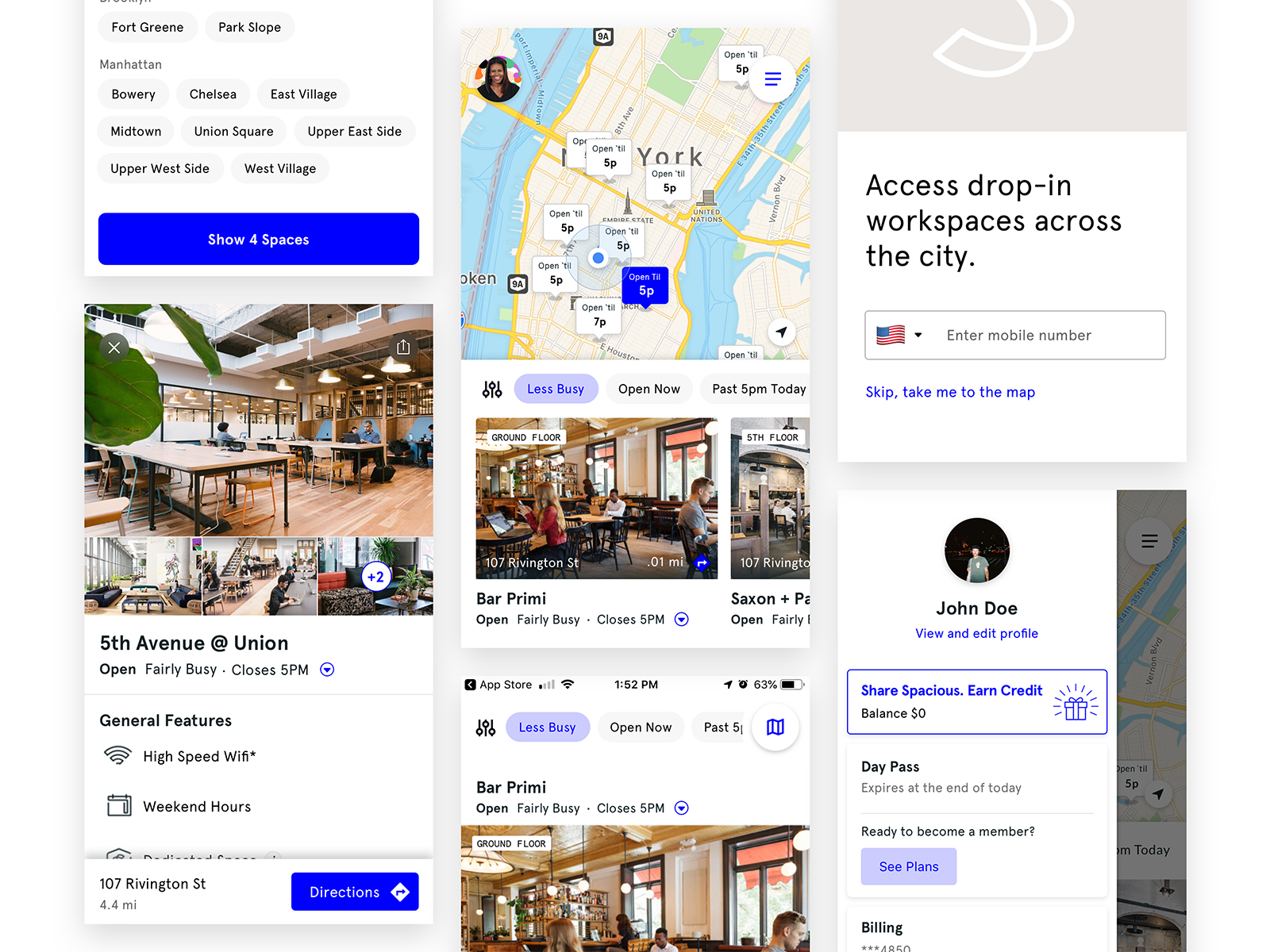This image appears to be a screenshot of a laptop screen displaying a travel or coworking platform's interface. At the top, there are oval-shaped buttons with the labels "Fort Greene" and "Park Slope." Below these buttons, a heading reads "Manhattan," followed by a list of neighborhood names, including Bowery, Chelsea, East Village, Midtown, Union Square, Upper East Side, Upper West Side, and West Village. 

Beneath this list is a large, blue rectangular button labeled "Show Four Spaces." Accompanying the button is a tropical-themed image that resembles a bar, indicative of a locale in the city, specifically noted as "Fifth Avenue at Union." 

To the right of the screen, there is a sidebar that reads "Access Drop-In Workspaces Across the City." This section includes fields to input a phone number and displays a user profile for "John Doe" along with information about day passes and billing.

In the middle segment of the screen, additional destinations and a drawn map are visible. There’s also a partial image at the bottom, which is cut off, but it includes the text "Ground Floor." The screen contains internet icons and navigation options, suggesting a versatile, user-friendly interface for exploring urban workspaces.